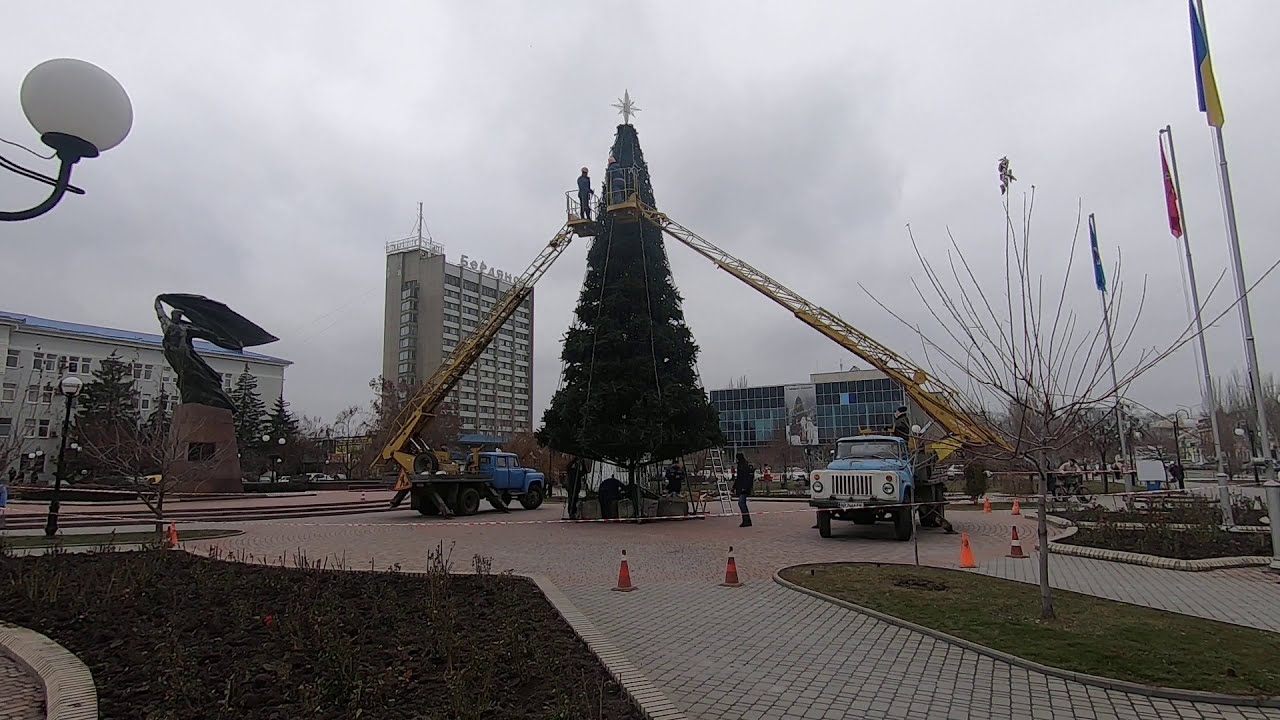In this image, taken during a gray, cloudy day, we observe a bustling urban square or city park showcasing the assembly of a large Christmas tree adorned with a star at its top. The scene features two blue trucks, each equipped with yellow cranes extending outwards at an angle, with workers in buckets meticulously placing ornaments and decorations on the tree. Surrounding the area are various safety measures, such as orange cones and caution tape, ensuring the space is secure. 

The ground is a patchwork of red brick walkways interspersed with greenery, framed by areas of grass and garden beds. Barren trees indicative of winter and tall poles holding flags—yellow and blue, red, and blue—add to the urban landscape. The backdrop includes a mix of architectural structures: a low-hanging white building, a high-rise, another modern glass-fronted building, and an apartment or hotel-like structure. A notable statue with a red granite base and bronze figure stands prominently to the side. Street lights and additional lamp posts dot the area, encapsulating the essence of a city center preparing for the festive season.